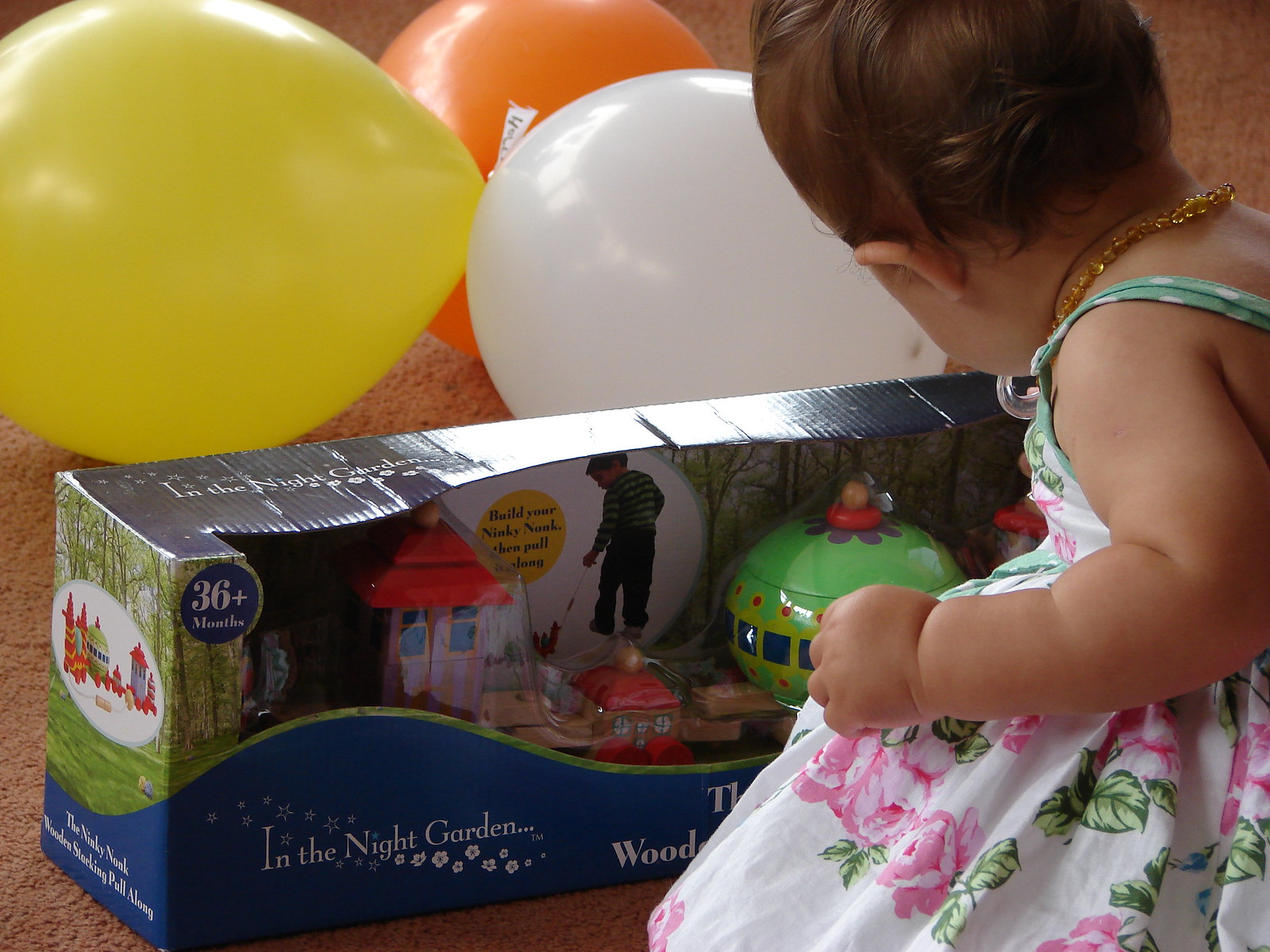In a cozy indoor setting, the photo captures a baby girl engrossed with a boxed toy in front of her. She is gracefully dressed in a white dress adorned with red flowers and green leaves, complemented by a delicate gold necklace around her neck. Her short brown hair frames her face as she bends down to touch the toy, a pull-along car with a green body and red top, nestled inside a blue box. The box is decorated with a green wave pattern and prominently features a logo reading "36+ months" along with "In the Night Garden" in the lower-left corner. Behind her, three vibrant balloons—a yellow, an orange, and a white one—add a splash of color to the scene, set against a backdrop of rich brown hardwood flooring.